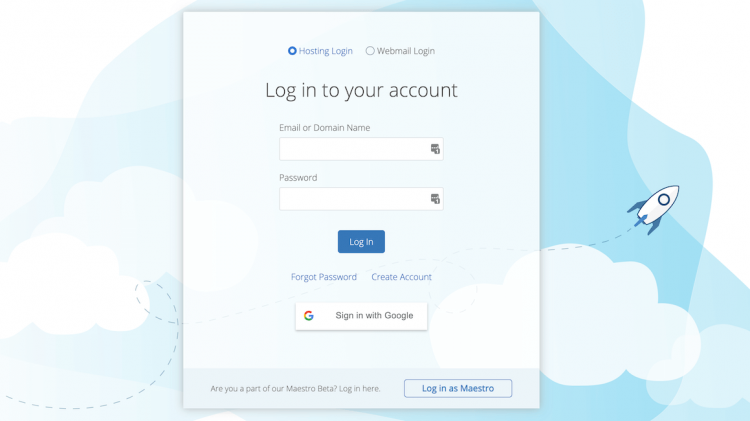The image presents a user interface for a login page with various elements distinctly laid out. At the top of the page are two options: the left button, highlighted in blue, is labeled "Hosting Login," while the right, bordered by a thin circle, is labeled "Webmail Login." Below these, a gray text prompts users to "Login to your account."

Further down, there are two fields for user input. The first field is indicated by gray placeholder text, "Email or Domain Name," and the second, labeled "Password," both awaiting user information. Beneath these fields lies a prominent blue "Login" button featuring white text.

Next, two blue links are presented: "Forgot Password" and "Create Account," positioned side by side.

Below these, a white button marked "Sign in with Google" is adorned with Google's colorful "G" icon on the left. A darker blue section underneath addresses users of the Maestro beta, inviting them to "Login here" using a button labeled "Login as Maestro," outlined with a blue border.

The background features a stylish design with various blue shapes and an illustration of a spaceship on the right, soaring above a cluster of clouds below.